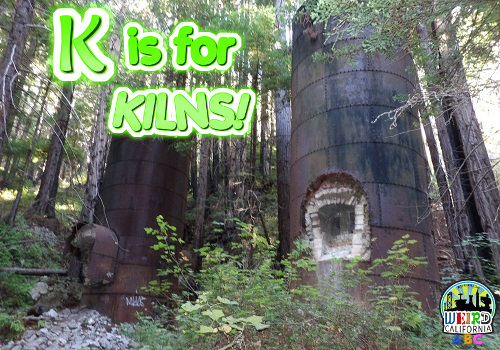This photograph captures a rustic scene featuring two weathered metal structures, reminiscent of industrial kilns, standing tall amidst a verdant forest backdrop on a hilly slope. The large and smaller riveted metal towers, appearing aged with a rich patina, sport brickwork or oven-like facades at their bases. The larger structure hints at a central archway, possibly an entry point. Beneath the oven facing on the lower left side, a pile of stones or debris can be seen. Surrounding the structures is a scatter of gravel and dirt, intermingled with dense greenery comprising bushes, weeds, branches, and leaves against a backdrop of towering trees. Text overlaid in neon lime green bubble font reads "K is for Kilns" at the upper left corner, lending a whimsical touch to the image. The lower right-hand corner is marked with the "Weird California" logo, adding a unique signature to the photograph.